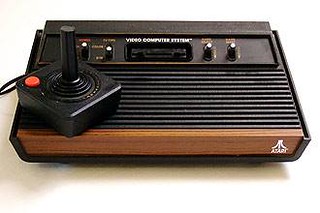This is a detailed product photograph of a classic Atari video game console, taken against a white background with shadows casting towards the bottom left. The console features a light tan faux wood front panel with a white Atari logo in the lower right corner. The main body of the console is predominantly black with ribbed stripes running across the top. The upper portion houses controls including four toggle switches and two knob controllers, each marked with a white dot. In the middle of this area, there is a prominently visible slot for game cartridges, labeled with the white text: "VIDEO COMPUTER SYSTEM."

Additionally, the image includes a classic Atari joystick controller. Positioned to appear as a diamond, it has a rectangular black base with concentric rings around the centrally protruding joystick, mimicking the gear shifter rings found in a car. An orange button is located in the upper left corner of the controller.